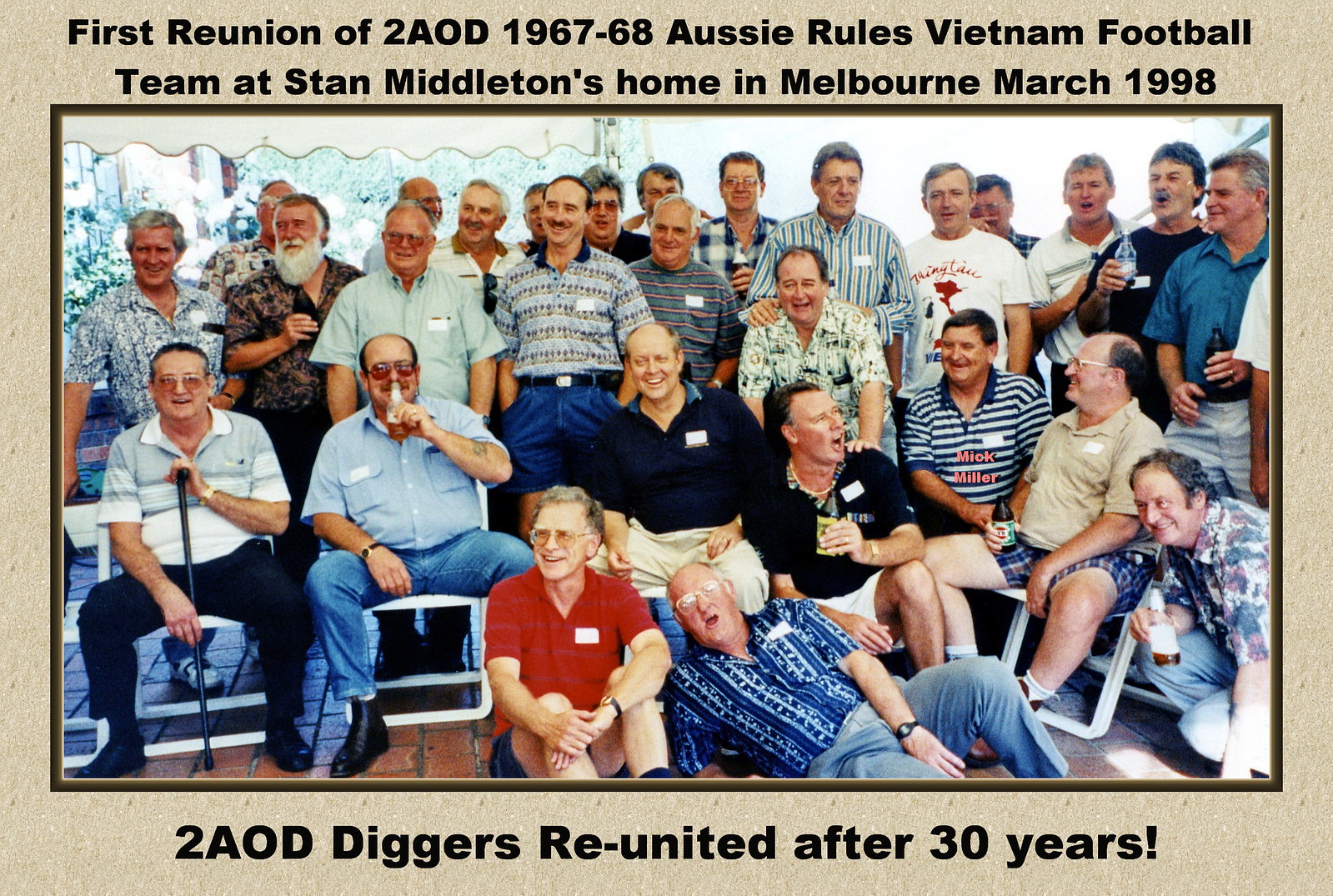The photograph captures a vibrant reunion of elderly gentlemen, members of the 2AOD 1967-68 Aussie Rules Vietnam Football Team, taken at Stan Middleton's home in Melbourne in March 1998. The men, approximately 30 in number, are dressed in slacks and short-sleeved shirts, which suggests warm weather. Their attire is casual, with some donning sunglasses or eyeglasses and a few gripping canes. Gray beards are common among them, highlighting their age. While some sit in white chairs and others on the ground, a row of men stands at the back, creating a layered and dynamic composition. The light brown border around the photograph contains black text at the top, reading "First Reunion of 2AOD 1967-68 Aussie Rules Vietnam Football Team at Stan Middleton's home in Melbourne, March 1998," and at the bottom, it states "2AOD Diggers, Reunited After 30 Years." Many of the gentlemen are smiling, holding bottles of beer, and appear genuinely happy to be in each other's company again after three decades.